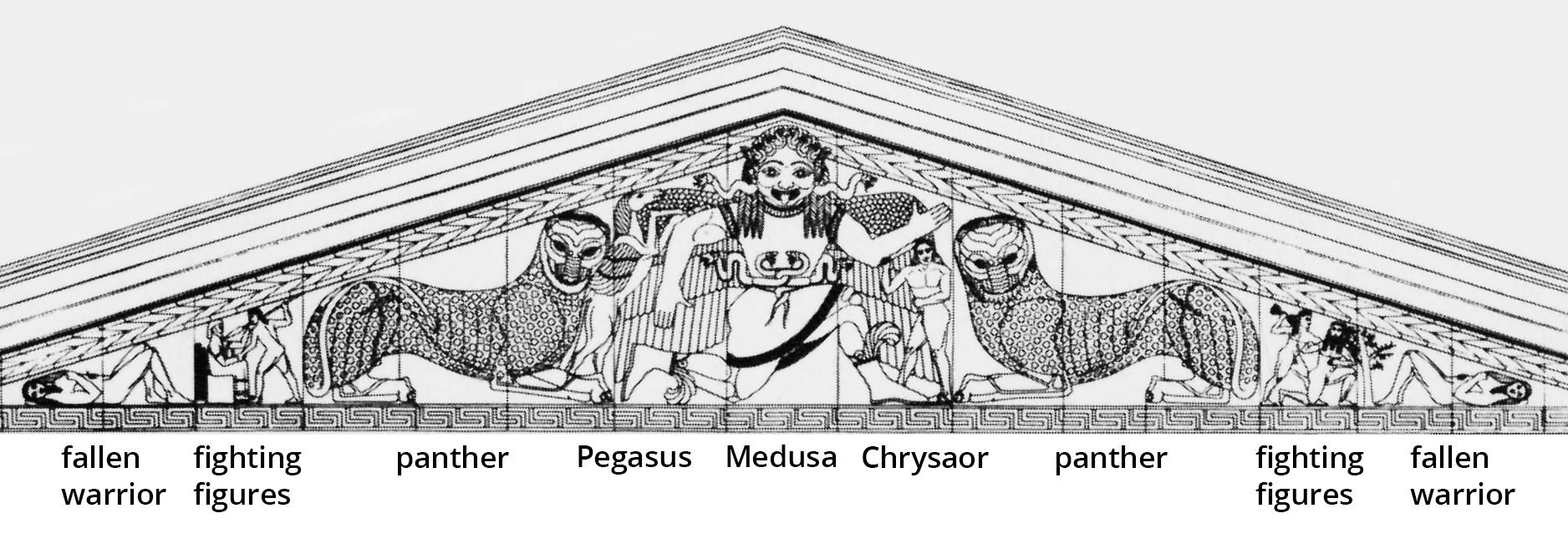This detailed black-and-white line drawing resembles a long, skinny rooftop centered at the top of the image, drawn in a flat Grecian style reminiscent of ancient pottery. The pyramid-shaped image, divided symmetrically from the center outwards, is filled with mythological figures and scenes. 

At the top-center of the pyramid stands Medusa with her tongue sticking out, flanked by her iconic wings and crowned head. To the right of Medusa, we see figures labeled as Chrysaor, possibly a mythological entity. Moving further right, there is a stylized panther with almond-shaped eyes and a dark patch around its nose and mouth, a depiction of fighting figures with one man stabbing another, and a fallen warrior lying on his back with his knees up.

Mirroring these scenes on the left side, the sequence is repeated with a fallen warrior, fighting figures, the stylized panther, and Pegasus, the winged horse from Greek mythology. The visual symmetry and intricate details offer a compelling depiction of Grecian mythology, with each figure carefully named and positioned to balance the composition elegantly.